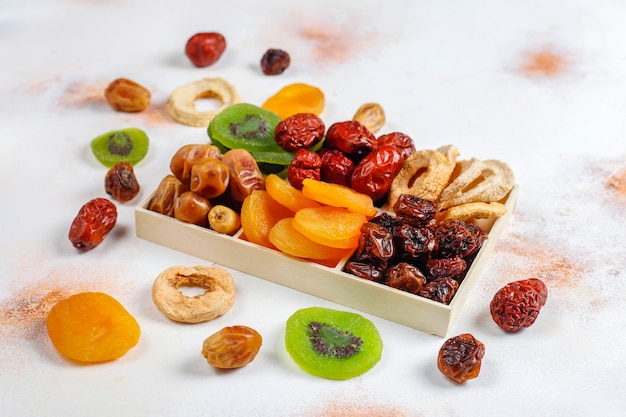The square, full-color photograph depicts a meticulously staged arrangement of dried fruits and nuts on a light blue tablecloth with a red design. Central to the image is a rectangular wooden box with three compartments, each filled with a variety of vividly colored dried fruits. Surrounding the box are additional loose pieces of dried fruit. The box features dried apricots (bright orange), sliced kiwis (green with black seeds), and various other dried fruits such as prunes (dark brown) and dates (reddish-brown). Beige, onion ring-like items are also visible. Sprinkles of seasoning are scattered across the background, adding texture to the scene. The overall composition showcases a visually appealing assortment of dried fruits, making the photograph both colorful and texturally rich.